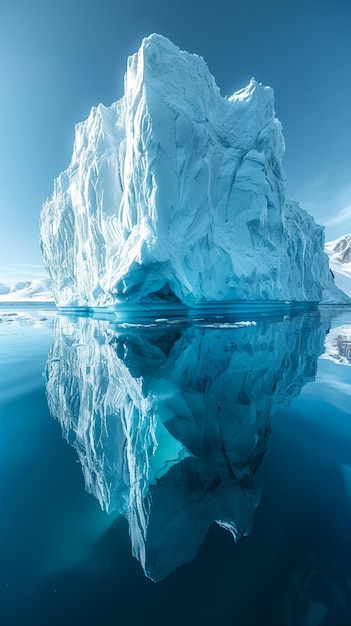This color photograph captures a stunning scene dominated by a giant iceberg emerging from a calm, pristine ocean that reflects the iceberg almost perfectly. In the lower half of the image, the water, varying in shades of blue from darker at the bottom to lighter towards the middle, mirrors the iceberg's detailed structure. The iceberg itself is bathed in light from the left, showcasing a contrast of whites and blues—white where the sunlight hits directly and a deeper blue on the shaded right side. The front of the iceberg intriguingly resembles the bow of a ship, with a small cave-like formation at its base, adding to its grandeur. Surrounding the iceberg, there are hints of either land or additional ice formations, presumably covered in snow. The backdrop features a vast blue sky adorned with some wispy white clouds near the horizon. This serene and reflective setting hints at a strongly illuminated environment from the left, casting an ethereal glow over the landscape.